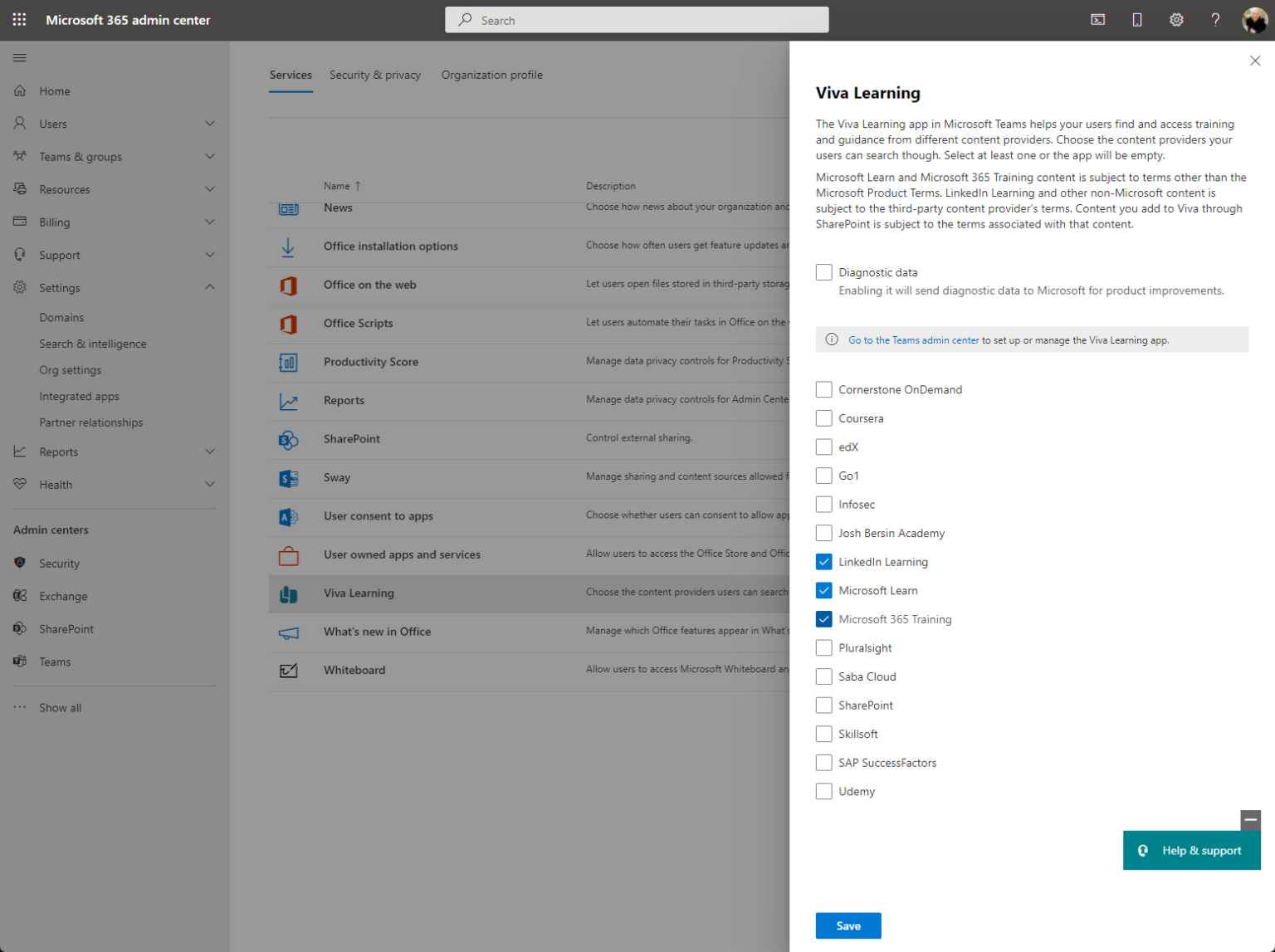A detailed caption for the described image:

"Screenshot of the Microsoft 365 Admin Center highlighting various administrative sections such as Services, Security & Privacy, and Organization Profile. The right pane showcases information about the Viva Learning app in Microsoft Teams. The pane explains that Viva Learning assists users in finding and accessing training and guidance from multiple content providers. Administrators are prompted to select at least one content provider; otherwise, the app will remain empty. Content choices include Microsoft Learn and Microsoft 365 training, which are subject to specific terms different from standard Microsoft product terms. Additionally, LinkedIn Learning and other third-party content follow their respective providers' terms. Content added through SharePoint adheres to associated terms. The option to enable diagnostic data, currently unchecked, includes a note that enabling it would send diagnostic data to Microsoft to improve products."